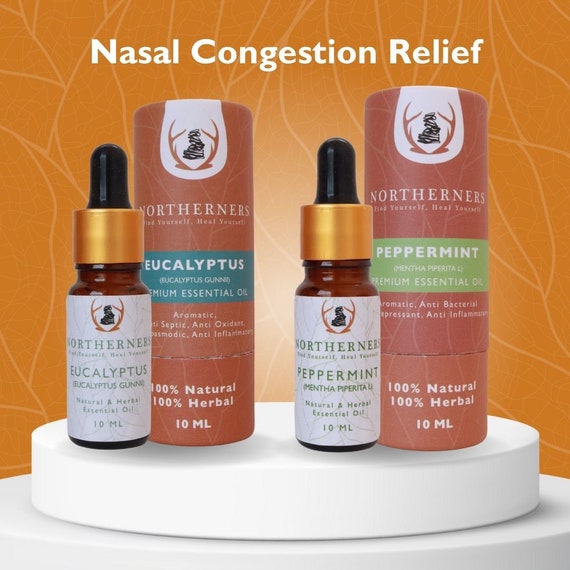This advertisement showcases two nasal congestion relief products from the brand Northerners, prominently displayed against an orange background with bright lines. At the top center, the text reads "Nasal Congestion Relief." The products, packaged in small dropper bottles, are each 10 milliliters in size and made from 100% natural and 100% herbal ingredients. The product on the left is a eucalyptus premium essential oil, while the one on the right is a peppermint premium essential oil. Both bottles feature a white label with the specific odor labeled, a gold cap, and a black tip. The items are placed on a white display dish, with the bottles positioned next to their respective packaging. The packaging highlights the product details and the Northerners logo.